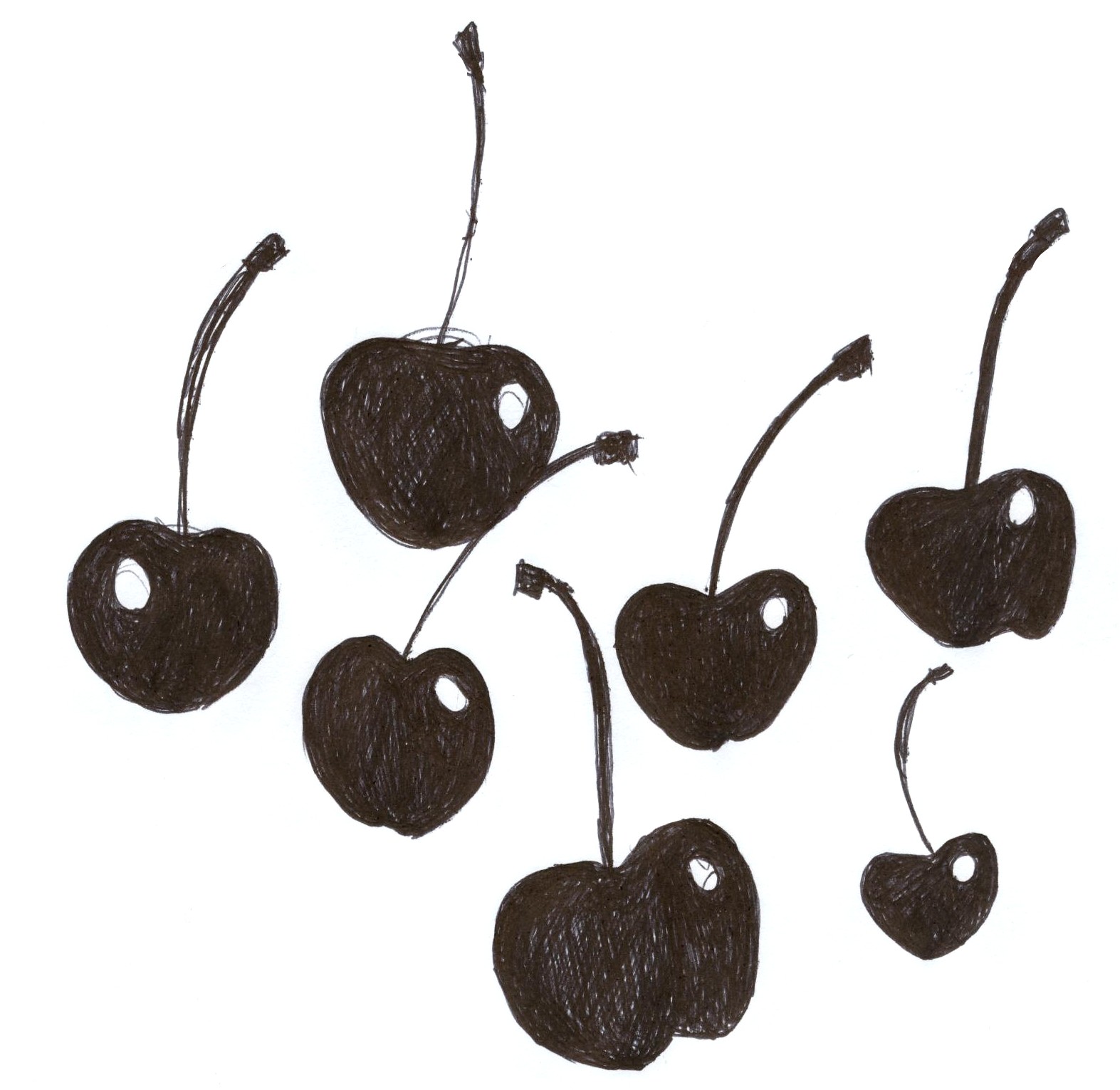The image depicts a detailed sketch of seven black cherries drawn with what appears to be a black marker or charcoal pencil. Set against a stark white background, the cherries vary in size, with two of them standing out as the largest. Each cherry features a distinct stem that curves gracefully, ending in a thicker, blackened point where it would have been detached from the branch. A small white highlight on the upper right side of almost all the cherries indicates a light reflection, adding to the overall realism of the sketch. The cherries are shaded in dark, but there are subtle gaps where the texture of the paper shows through, enhancing the intricate detailing of the drawing. The arrangement of the cherries is somewhat random, clustered together without forming a neat row, and their stems curve in different directions, adding a lively dynamic to the composition.